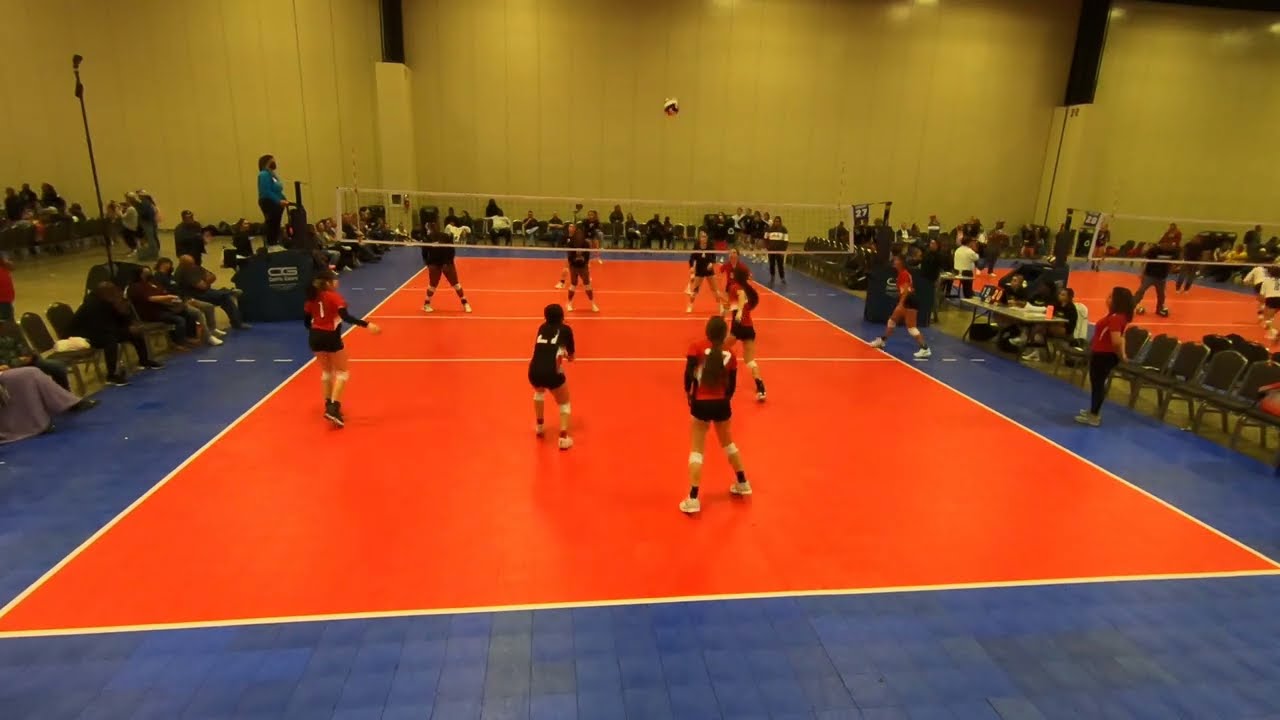The photograph captures an indoor arena with two volleyball courts, featuring a vibrant scene of girls playing volleyball. The primary court in focus is a bright orange with white boundary lines, surrounded by a blue floor made of square tiles. On this court, a team in red jerseys and black shorts is prominently shown in the foreground, with one player in an all-black outfit. The opposing team in the background wears all-black jerseys and shorts. 

A volleyball hangs in mid-air above the court's center, while spectators fill plastic chairs along the left side, indicating a lively audience possibly comprising parents, friends, and fans. The left side also features a platform for a judge overseeing the game progression, along with other judges in red shirts stationed at the court's edge. On the right, another partially visible orange court hosts more players, though this scene is less clear and partly obstructed. Between the two courts, a table with two seated individuals likely serves as the judging or scoring area.

The arena's walls are a tan or light greenish-yellow color, suggesting a gym-like environment. The overall atmosphere is bustling and dynamic, capturing both the intense gameplay and the supportive presence of spectators.